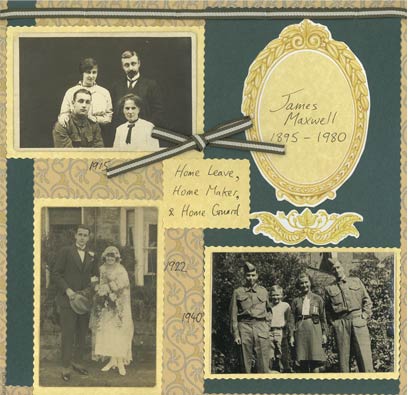This square image appears to be the cover of a scrapbook chronicling the life of James Maxwell, who lived from 1895 to 1980. The scrapbook cover features a collection of old-fashioned black-and-white photographs and inscriptions that narrate significant events in Maxwell's life.

In the top left corner, there is a family photo from 1915 depicting four people: an adult couple, a young man, and a young woman. Below this, in the bottom left corner, is a slightly out-of-focus wedding photo of a man and a woman, dated 1922. The bottom right corner contains a 1940 photograph showing two soldiers in uniform along with a young man and a young woman.

In the top right corner, accompanying a meter motif, the text reads "James Maxwell, 1895 to 1980." The center of the scrapbook cover bears the titles "Home Leave, Homemaker, and Home Guard," suggesting themes that may be elaborated within the album. A ribbon tied into a bow adds an elegant touch to this detailed and nostalgic compilation of James Maxwell's life journey.